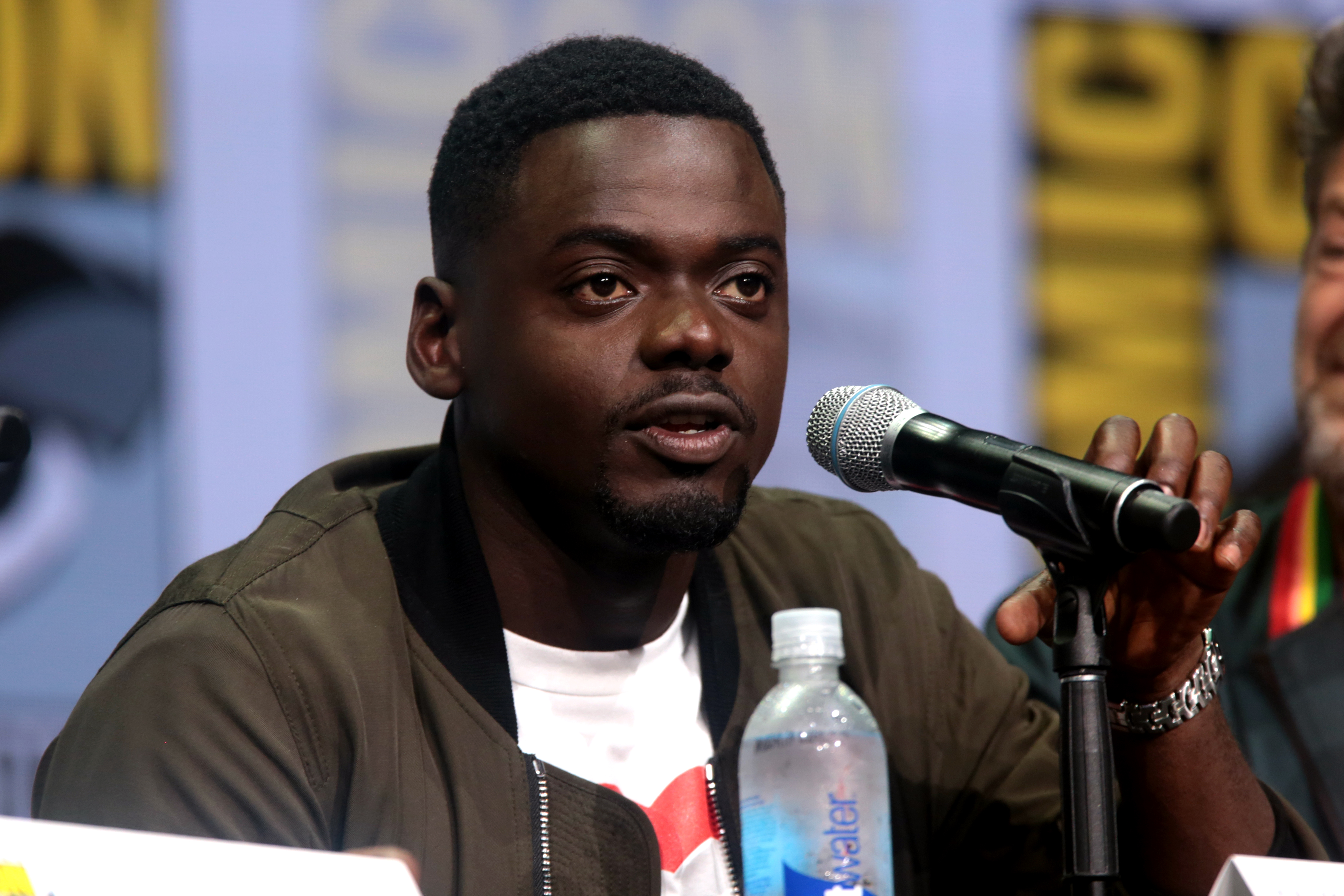The image features a black male seated at a conference panel, positioned behind a microphone mounted on a stand. He is dressed in a dirty green bomber jacket with a black collar over a white t-shirt that has red elements. The man has short black hair, a black goatee, and slightly bloodshot eyes. His mouth is open, suggesting he is speaking, while his left hand is reaching out towards the microphone. He is wearing a silver, potentially stainless steel, watch on his wrist. In front of him are a water bottle with a white cap and several name tags with illegible names. Another man, dressed in a black top and sporting a beard, is seated to his right, looking in his direction. The background features a white wall with out-of-focus red text, likely the Comic-Con logo, and the outline of an eye on the left side of the image.